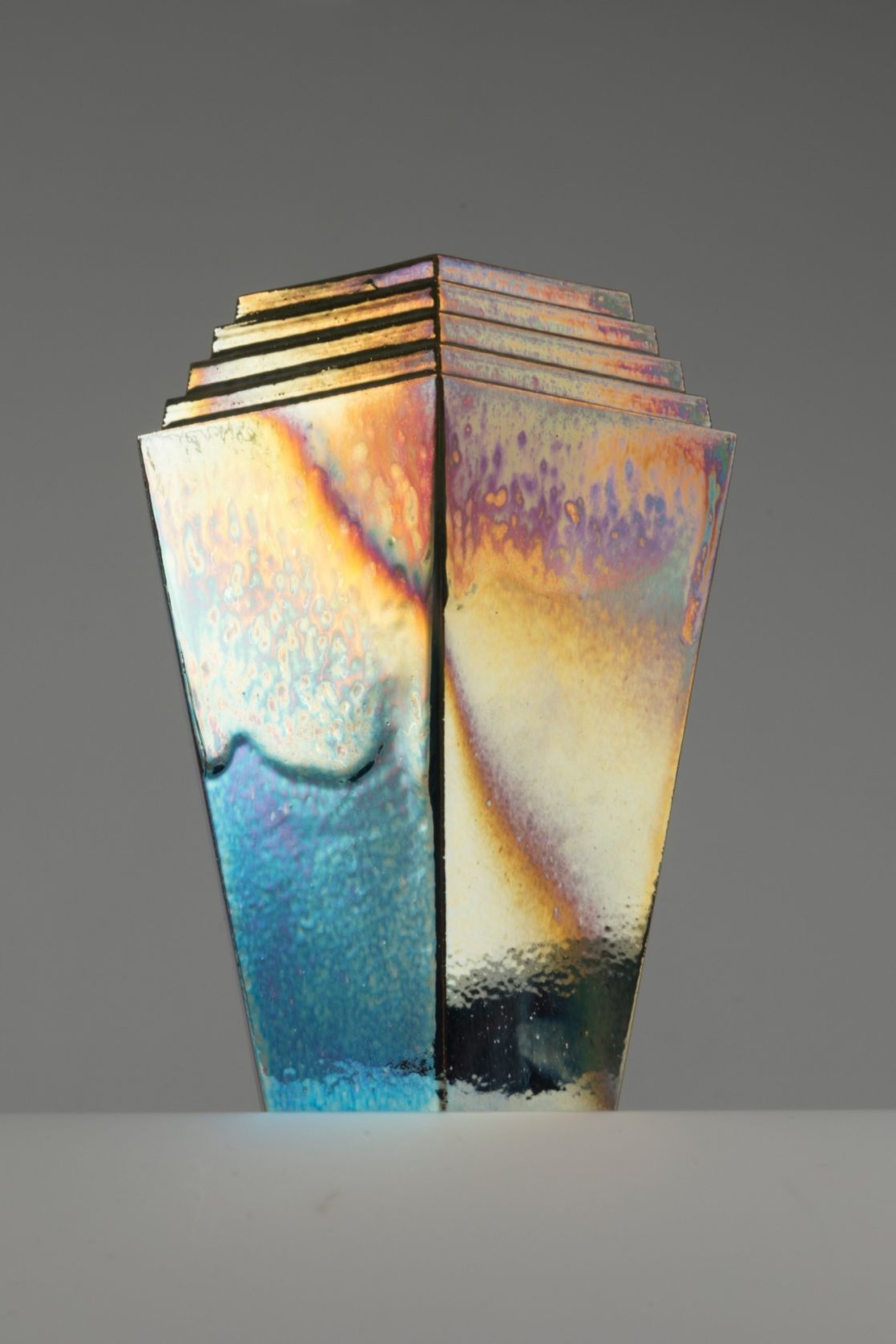The image is a vertically aligned rectangular photograph depicting an unusual, multi-colored vase or metallic object against a solid dark gray background that transitions to a lighter gray at the bottom. The main object has a distinctive angular design with four sides, of which two are visible and separated by a black line. The left side of this object features a textured blue bottom and a textured upper portion in shades of yellow and brown. The right side has a black area at the bottom, followed by yellow in the middle, and a vibrant blend of purple, orange, yellow, and blue at the top. The object is structured in a tiered manner akin to steps that become progressively smaller towards the top, reminiscent of stacked square cups or the upper part of a lamp post. The entire object has a metallic, shiny appearance, with its colors merging smoothly into each other, creating a unique tie-dye effect. The object is positioned against a gray background that serves as both the wall and the surface it rests on.